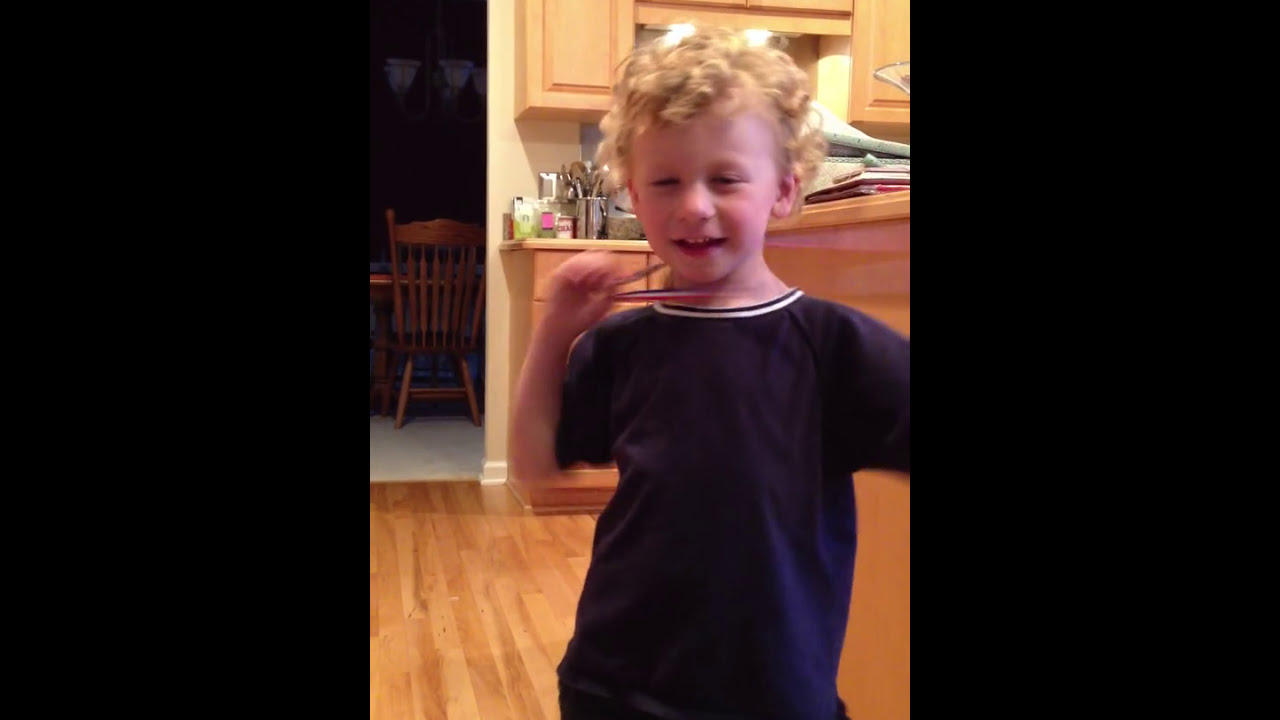The image is a photo of a young boy, captured in a three-panel layout with black borders on the left and right. The middle panel, which is much larger, showcases the boy standing and smiling with his mouth open, eyes squinted, and showing his top teeth. He has short, curly blonde hair and is wearing a blue short-sleeved shirt cut off at the waist. Around his neck, he has a lanyard that is red, white, and blue, which he holds up in his right hand. Though slightly blurred, it seems he is waving or displaying a medallion. His left arm is out of the frame. The background reveals a kitchen with light-colored hardwood flooring, cabinets, and a cluttered counter with various utensils and containers. Further back, an entryway leads to another room where a brown wooden chair is visible. The boy appears to be celebrating, capturing a moment of cheerful motion.